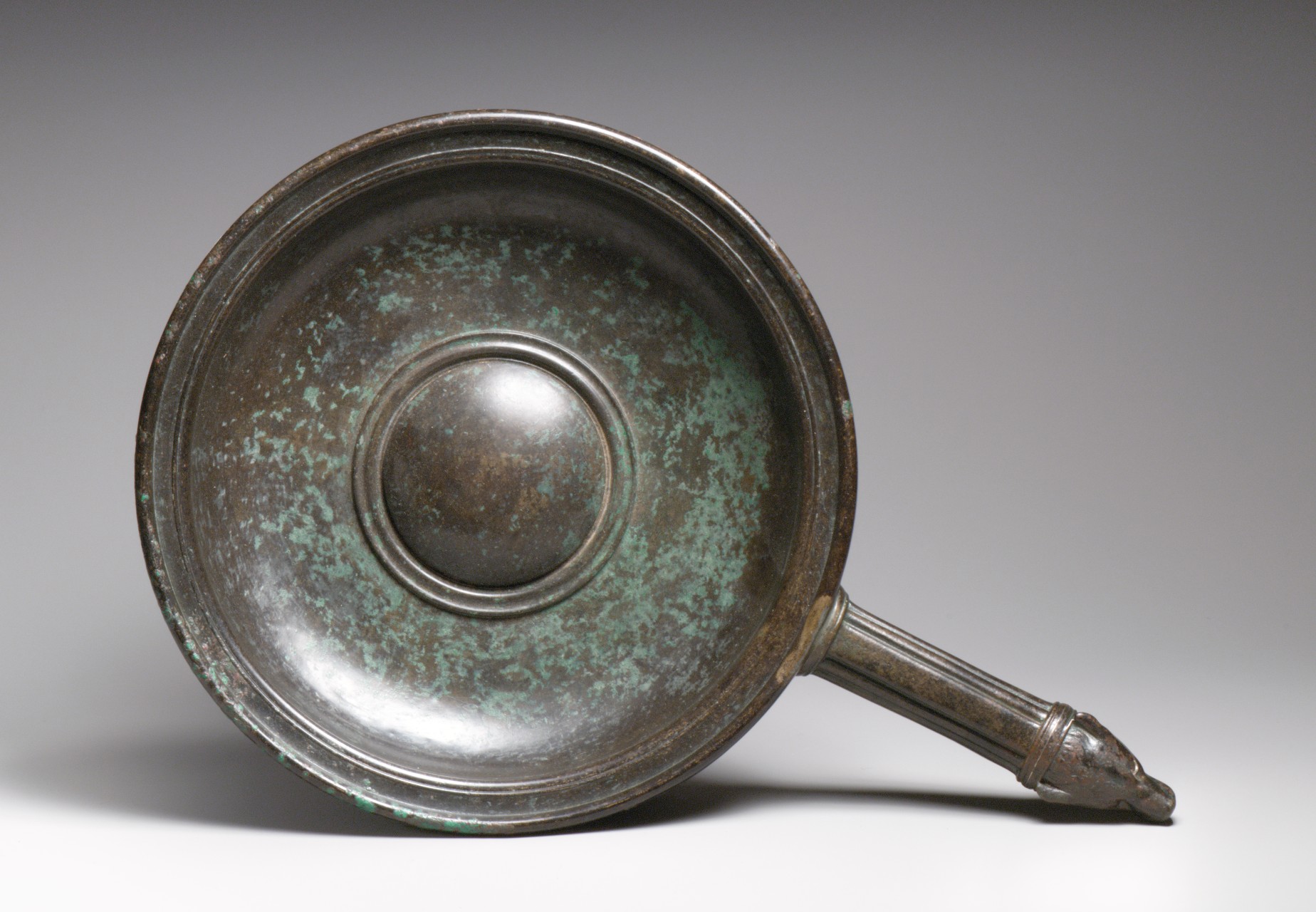This is a meticulously staged, full-color, close-up photograph of an aged, tarnished frying pan-like artifact, depicted indoors against a predominantly gray background that fades to almost white in the lower right corner. The artifact’s circular body appears worn, primarily copper-colored with patches of green oxidation that resemble tarnished grass. A prominent large circle in the center of the pan is encircled by a smaller raised copper band. The wooden handle of the artifact is ornate, culminating in an animal head carving at its end. The overall image, capturing this ancient, dull silver and copper-hued pan, highlights its rough texture and intricate details, leaving its exact purpose open to interpretation.